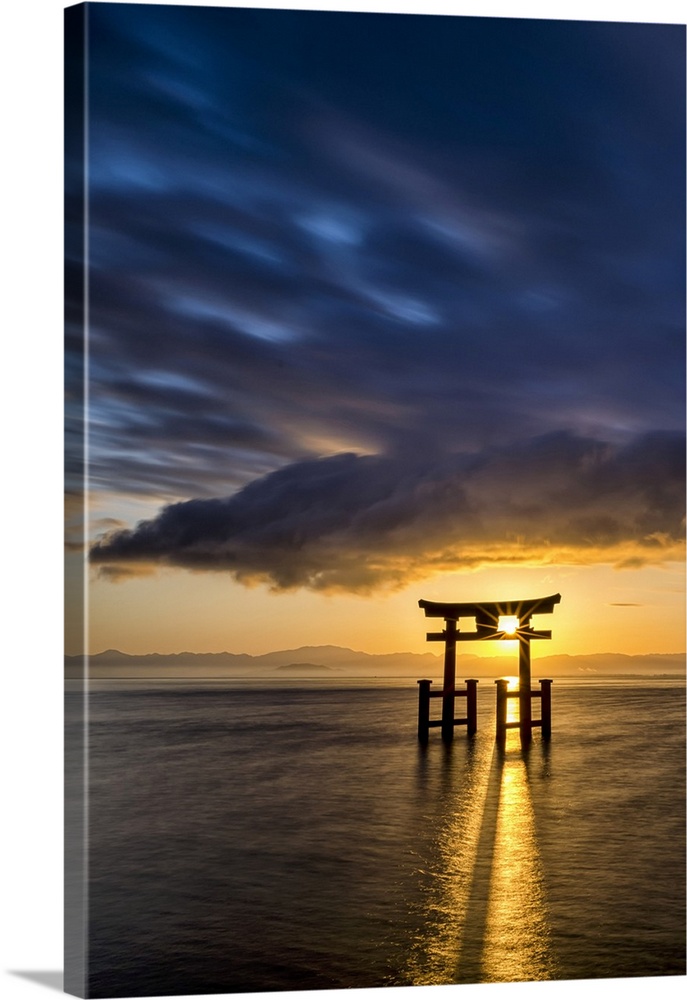The image portrays a serene sunset scene over a lake in Japan, captured in either a highly detailed painting or a photograph. Dominating the foreground is a torii gate, its intricate wooden frame silhouetted against the vibrant sky. The sun casts warm, golden-yellow rays through one of the holes in the torii gate, illuminating the sky with a beautiful gradient of orange and yellow hues. Heavy, navy blue clouds loom above, their tops dark gray while their bottoms catch a golden light. This creates a dramatic yet peaceful contrast. The lake beneath reflects the brilliant sunlight and shimmering sky, with gentle ripples indicating a slight breeze. There is also a faint hilly shoreline in the distance, enshrouded in a light fog, adding to the mystical allure of the image. The overall composition exudes tranquility and natural beauty.